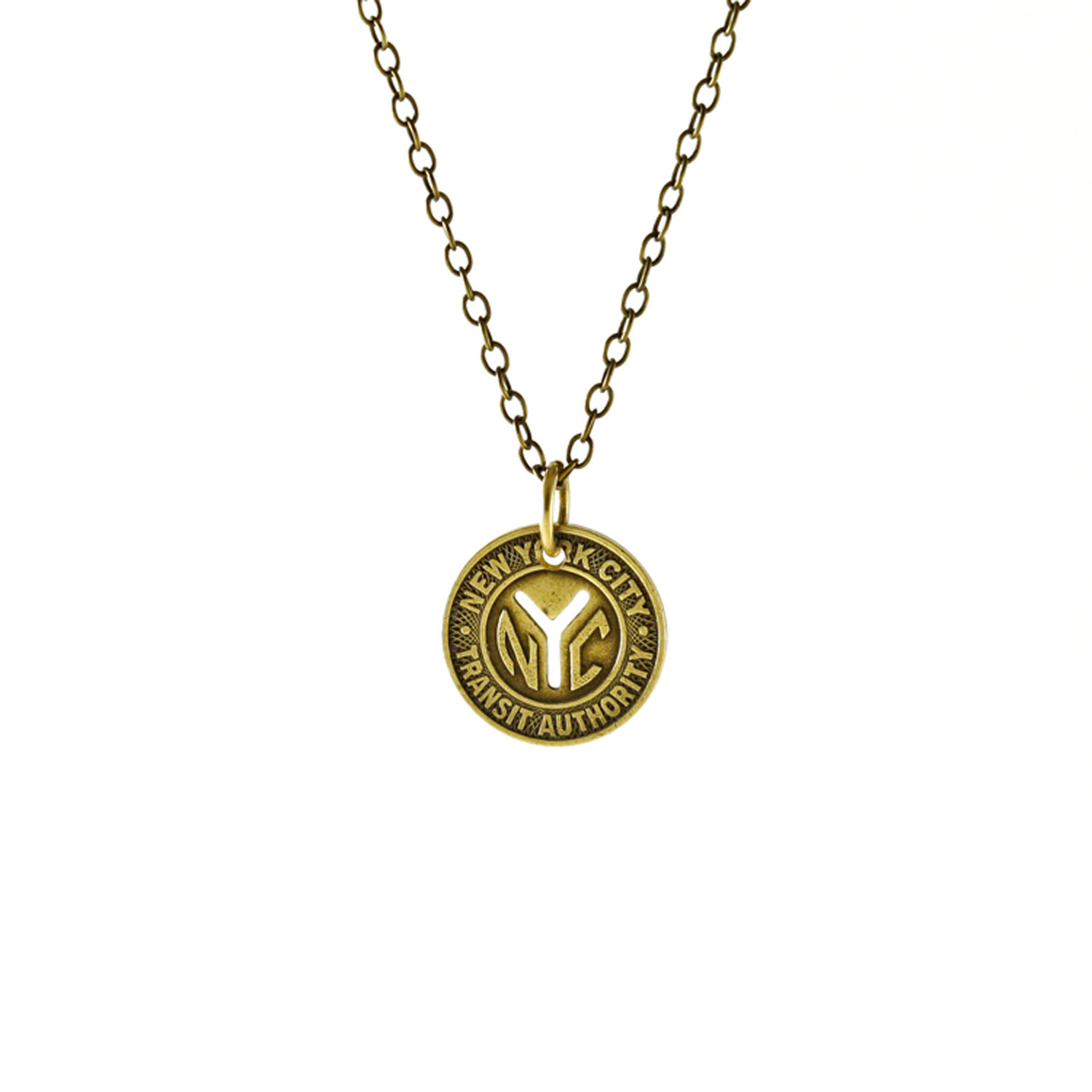This image showcases a gold chain link necklace featuring a pendant with intricate details. The necklace's chain, visible for a few inches above the pendant, suspends a small gold hoop that connects to a round, brass-colored metal pendant. The pendant is inscribed in a curved fashion with the words "NEW YORK CITY" at the top and "TRANSIT AUTHORITY" at the bottom, both in capital letters. The center of the pendant prominently displays the letters "NYC," with the "N" and "C" in gold, and the "Y" in white. The overall design combines elements of gold and brass tones, creating a harmonious and elegant piece of jewelry.